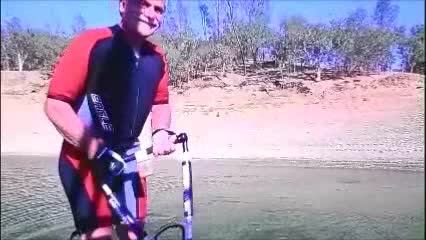In this image, an older man with a white mustache and beard stands in a calm, rippled lake, wearing a blue flotation life vest over a tight, short-sleeved outfit that combines red and blue shades, resembling a bathing suit or biking shorts. The man is gripping handles of an unseen water device, possibly with handlebars and a frame that might be purple and yellow. Below him, the lake water shows clear ripples, leading to a nearby shore. The shore transitions from white sand to reddish-pink sand or rocks, ascending into a tree-lined horizon. The tall green trees, some sparse with leaves, contribute to the tranquil scene under a crystal-clear blue sky, devoid of clouds. The man's knee appears bent on something, hinting at a dynamic stance, and shadows play across his figure, completing the detailed, serene lakeside scene.